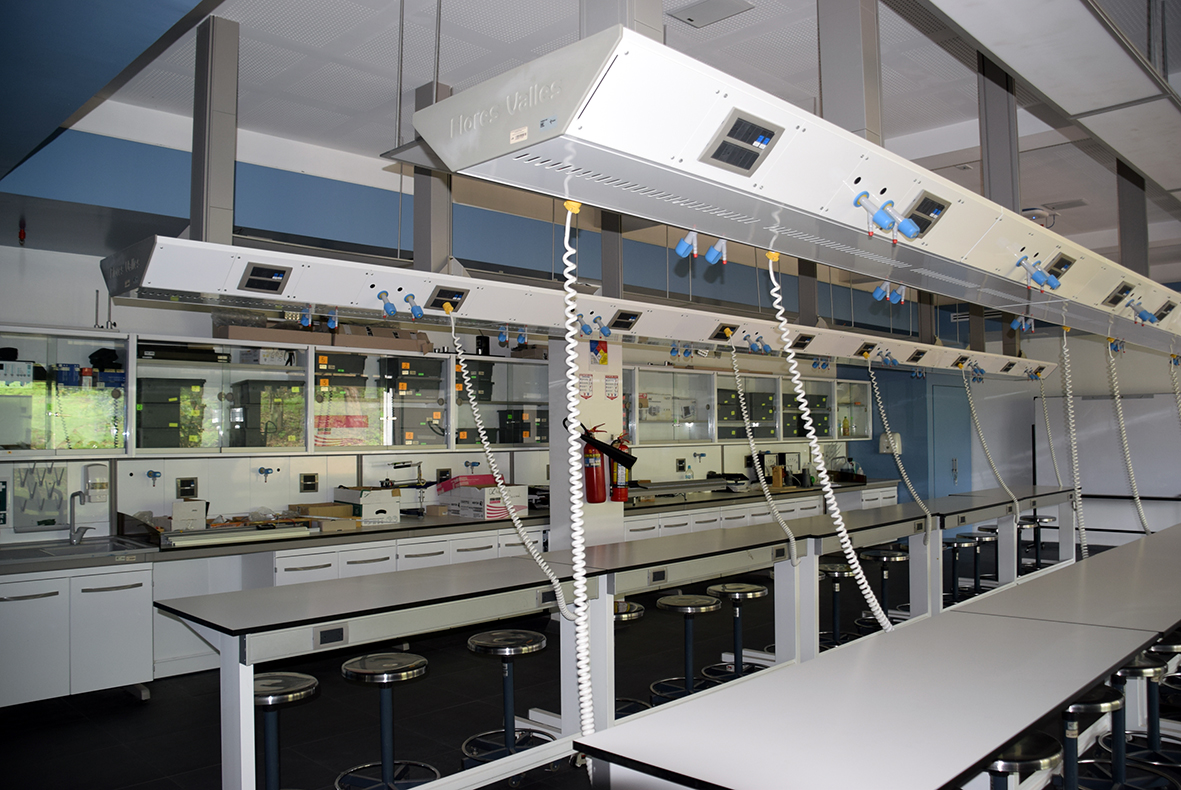This interior photograph showcases a large laboratory with tall ceilings, highlighting a meticulously organized and modern workspace. The room features multiple long, white and gray countertops or workstations lined with rows of round, stainless steel stools without backs, each equipped with a chrome-like circular ring for foot support and swivel functionality. Overhead, various devices hang from a coffered ceiling painted blue with a white center; these devices are rectangular and metal, with white coiled cords or tubes descending from them, resembling telephone cords. Towards the far end of the lab, there are high glass cabinets with sliding doors used for storage, clear cabinets holding boxes, and multiple sinks integrated into white laminate cupboards and stainless steel basins. Additional elements include a blue door, a whiteboard attached to one of the benches, and two fire hydrants mounted on a white column. The comprehensive layout and structured design suggest a high-functioning, educational or experimental setting.